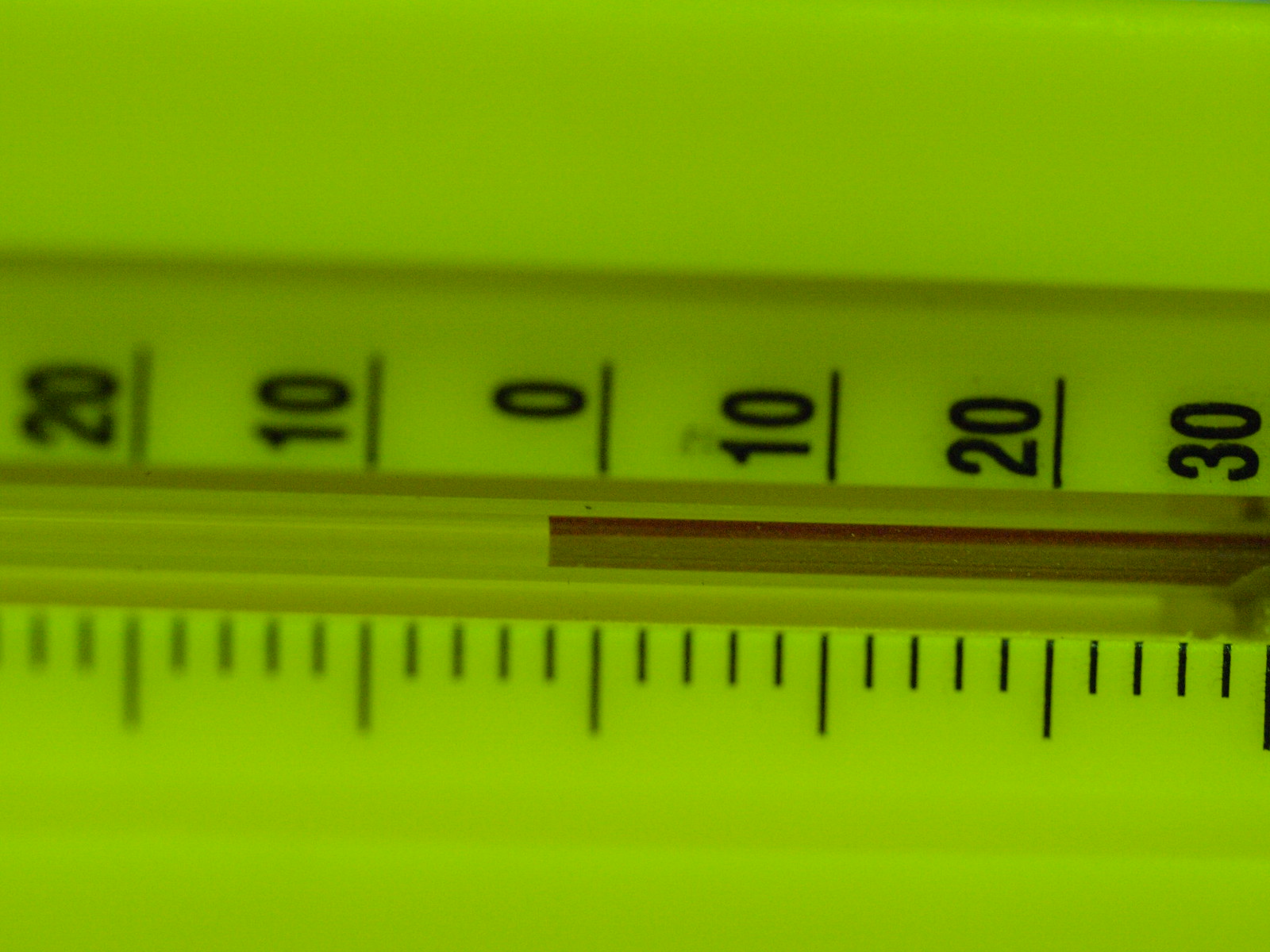The image features a thermometer placed on its side, suggesting the picture might be rotated 90 degrees counterclockwise. The thermometer's scale starts at 20 at the top, followed by 10, 0, and then descending to -10, -20, and -30. However, the negative symbols are not visible in this view. Along the scale, there are both longer and shorter marks; the shorter marks are spaced every two degrees. The thermometer shows a current temperature of 2, but there is no indication of whether the scale is in Celsius, Fahrenheit, or another unit. The liquid inside the thermometer is red, and the tube appears slightly pinkish. The background has a strong yellow tint which likely skews the color perception, indicating that the background is probably white and the tube is a standard glass. The overall lighting appears to be a light greenish-yellow, affecting the appearance of the thermometer and its surroundings.